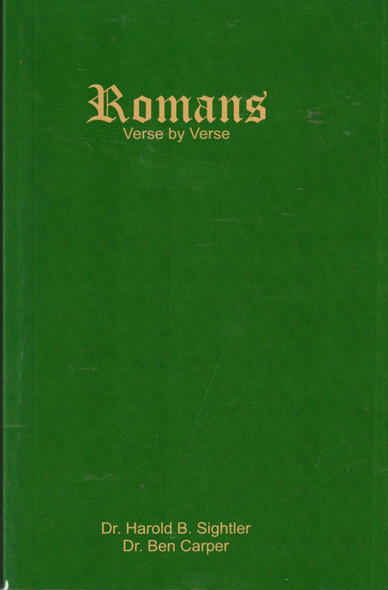The image depicts the front cover of a worn forest-green hardback book, filling the entirety of the rectangular frame, approximately four inches tall and two and a half inches wide. The book cover, exhibiting a faux leather texture with light wrinkling and superficial scratches, has a large noticeable scratch extending from the middle to the bottom. At the top, slightly off-center to the left, the title "Romans" appears in large gold letters with an old-fashioned, medieval font. Directly beneath it in smaller gold text, in plain English print, are the words "verse by verse." At the bottom, also off-center towards the left, is the name "Dr. Harold B. Seitler," with "Dr. Ben Carper" written underneath in the same smaller gold print. The cover shows signs of wear, including a rip near the bottom left-hand binding.